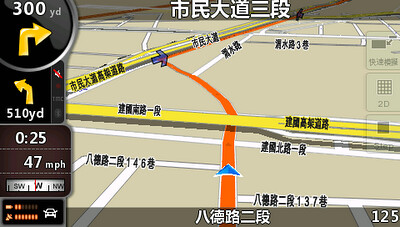A detailed still shot of a GPS device or navigation app screen, displaying route information in either Japanese or Chinese script. The map background is predominantly tan with white streets intricately woven throughout. The designated route is vividly marked in red, accented with blue directional arrows guiding the way. On the left side of the screen, a comprehensive panel provides various details: turn-by-turn directions, upcoming maneuvers, current time, driving speed in miles per hour, cardinal direction, and vehicle status. The visual information is clearly structured, despite the language barrier in the textual elements.